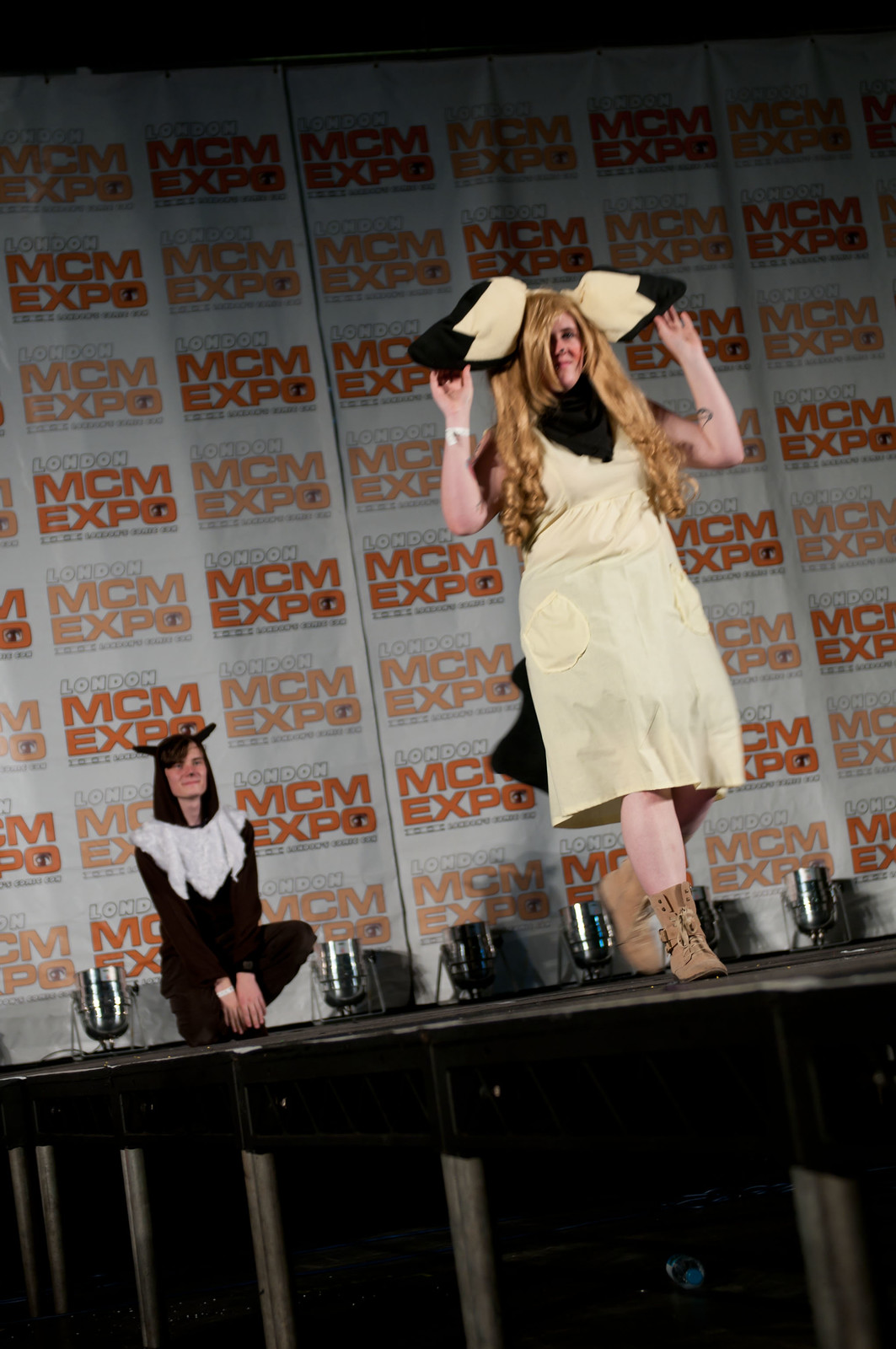In the image, an event resembling a fashion show or cosplay convention is captured from an audience's perspective at a tilted angle. Center stage, a woman stands confidently in brown boots and a knee-length, muslin-like white gown featuring circular pockets. She has long, auburn hair with curly ends and wears large, floppy ears or a bow, beige with black tips, on her head. Her hands lift the ears, and one foot is poised forward, suggesting an animalistic pose. Behind her on the stage, a crouched figure dressed in black is adorned with a white fur collar forming a V-shape and a hood with black ears. This person also appears to have a small black spot painted on their nose, suggesting an animal costume. The backdrop prominently displays the text "London" in white and "MCM Expo" in orange, repeated vertically. Support beams and spotlights further frame the stage, emphasizing the event's lively atmosphere.